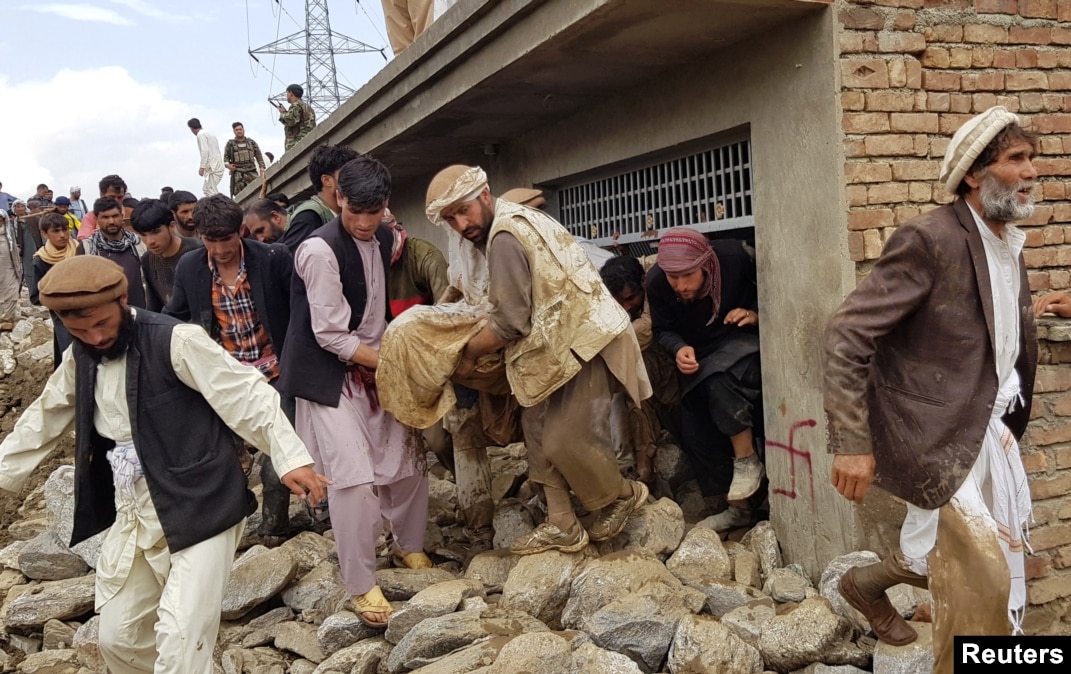This photo captures a large crowd of men, all adorned in traditional NWFP or Balochi garb, amidst what appears to be the aftermath of a disaster. The crowded scene shows these men actively navigating a rocky and rubble-strewn surface outside a damaged building. Two men are prominently seen carrying a body, wrapped in a white tarp stained with dirt, emerging from what seems to be a building with a pull-down gate, possibly a storefront. The air of urgency and solemnity is palpable as the men carefully step over large rocks and debris, which block the building's entrance. The building itself is marked with graffiti, potentially indicating it's been checked, and disturbing symbols, hinting at a hate crime. Amidst this organized chaos, power lines can be seen in the background, adding an element of normalcy to the harrowing scene. Additionally, some men stand on the roof of the building, while others mill around on the ground, reinforcing the sense of community in the face of adversity. The bottom right corner of the image bears the name of the news source, Reuters.